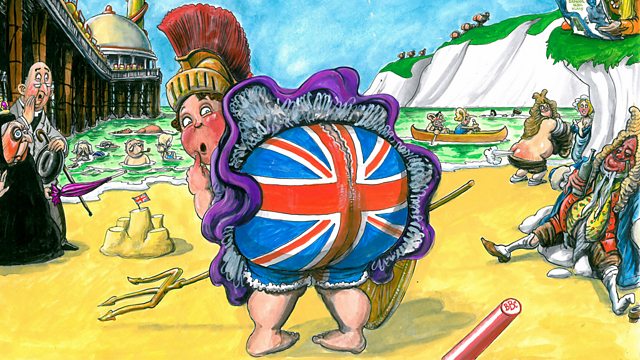The image is a detailed, cartoonish painting set on a vibrant yellow beach bordered by green water. A prominent jetty stretches out into the water. At the center of the scene stands a large, heavy-set man dressed in a comedic combination of Roman and British attire. He wears a gladiator-style golden helmet with a red mohawk crest and a purple skirt. The man is comically bent over, exposing his large, round backside adorned in torn underwear emblazoned with the British flag design – a blue background with a red cross and red X. His expression is one of shock, with wide eyes and an open mouth, and he holds a finger to his lips as if suddenly realizing his wardrobe malfunction.

Around him, various bizarre characters add to the humorous spectacle. To the right, a drunken man dressed in old-world British regalia, complete with a powdered wig, clutches a bottle. A few other characters populate the beach: one nearly nude figure in shorts seemingly in the midst of changing, and a startled priest or nobleman to the left, staring in astonishment at the scene. The entire image exudes a satirical tone, parodying British historical figures and Roman imagery in a whimsical beach setting.